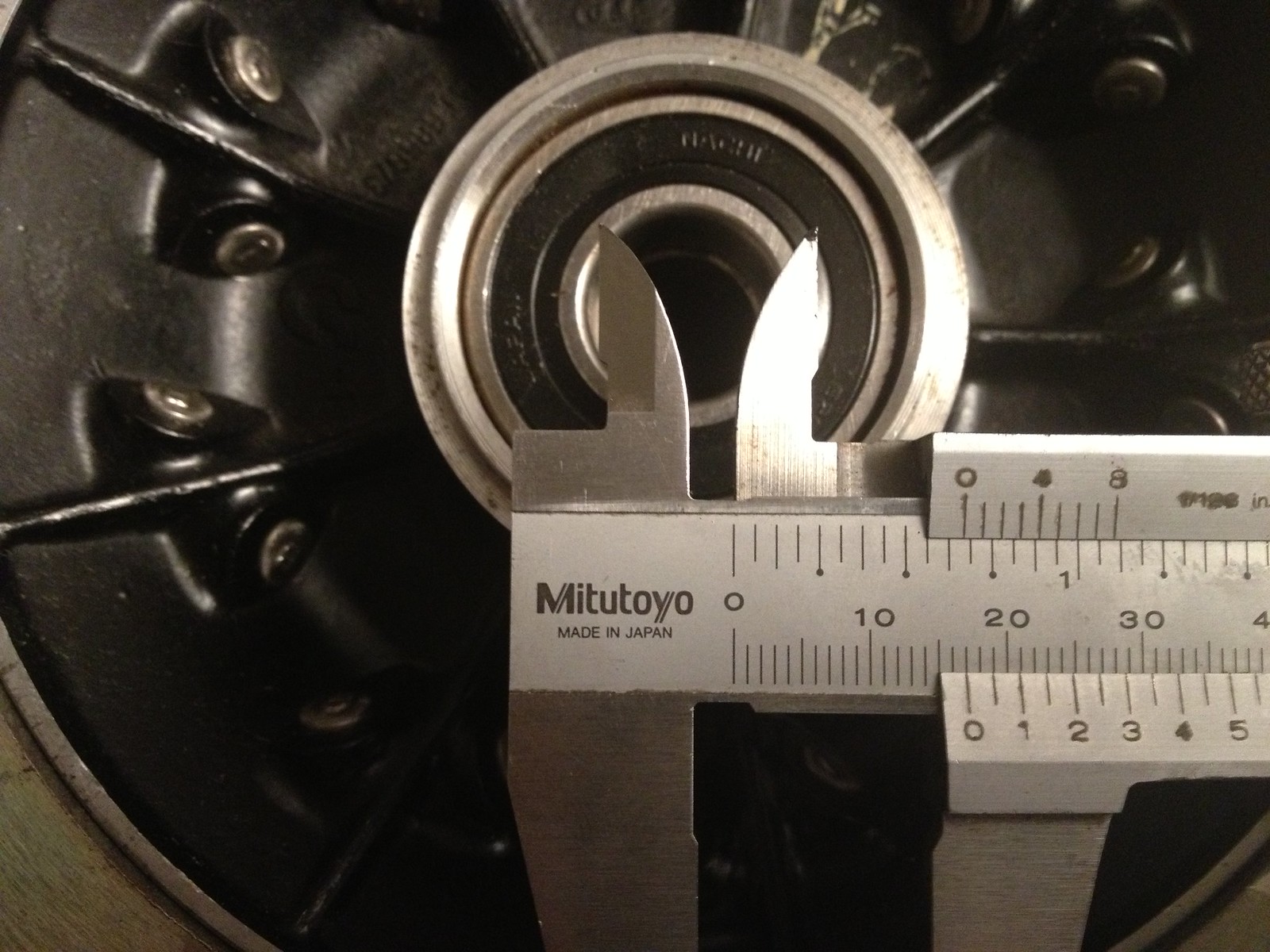The photograph depicts a detailed measuring device, identified as a ruler or scale, labeled "Mitutoyo, made in Japan." This stainless steel instrument appears to be specifically designed for precise measurements, possibly of diameters. The ruler features numeric markers from 0 to 40 and has two sharp, inverted blades or prongs at the top, likely for alignment with the object being measured. The background showcases what appears to be a car part, potentially a clutch plate or driver, characterized by its black surface and several screws. The car part includes a circular central section that might be the bushing, and the overall setup suggests the measuring tool is being used to gauge this segment's diameter accurately. The scene combines elements of silver and black metal, emphasizing the mechanical and precise nature of the equipment.